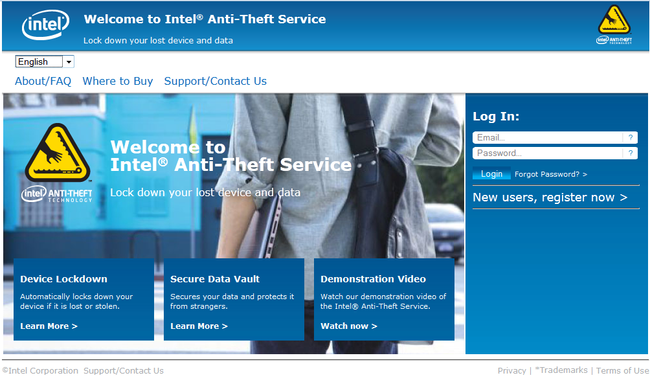The image showcases the Intel web page dedicated to its Anti-Theft Service. At the top, there's the prominent Intel logo set against a blue background with white text. Below the logo, a headline reads, "Welcome to Intel Anti-Theft Service. Lock down your lost device and data." 

The page is sectioned into various links such as "About/FAQ," "Where to Buy," and "Support/Contact Us." A notable feature is a logo displaying a black triangle with a black hand reaching towards a laptop, set against a yellow background.

A central login section prompts users to sign in with their email and password, alongside a blue "Login" button. Underneath, there’s an invitation for new users to register.

Information on the service is presented in three primary sections: "Device Lockdown," which describes how the service automatically locks down a lost or stolen device, accompanied by a white "Learn More" button; "Secure Data Vault," explaining how data is protected from unauthorized access; and a "Demonstration Video" section that encourages users to watch a demo, with a "Watch Now" button available for immediate viewing.

The predominant color scheme of the page is blue and white, consistent with the Intel branding. The background features an image of a person carrying a computer and a bag over their shoulder, suggesting mobility and the need for on-the-go security.